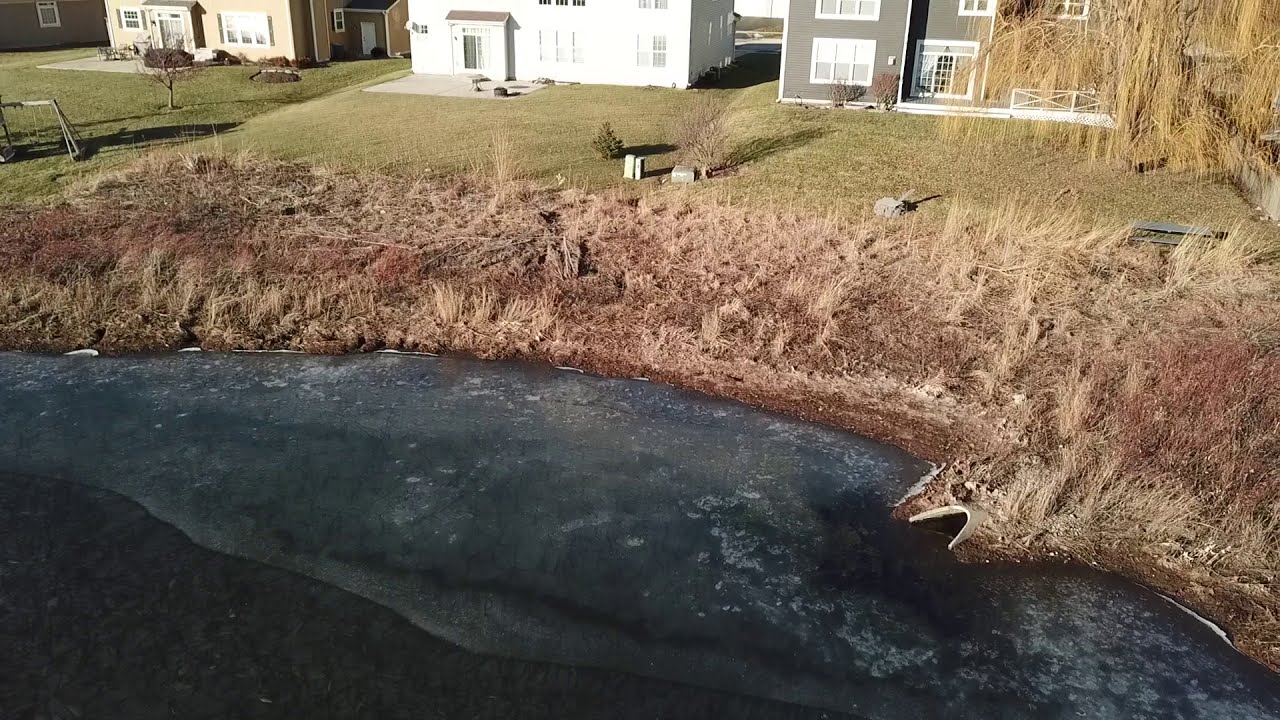This daylight exterior photograph, likely taken from a high vantage point such as a drone, showcases a small dark-colored pond nestled behind a row of rural homes. The pond, located at the bottom of the image, features a curved shoreline marked by dark red-brown earth and dotted with a variety of short, spiky, dead-looking plants, grasses, and other small vegetation. On the pond's right edge, there's a visible outflow of an underground pipe emptying water into it. 

Behind the pond, the landscape transitions from the untamed dirt shore to neatly mowed green lawns belonging to the houses. The series of homes includes a yellow house on the far left, a white house in the center, and a gray house with white trim on the right. Each yard features unique elements: the leftmost yard has a swing set and a tree, the center yard includes a small tree, and the rightmost yard has a barren tree and a bench area near the weeds.

Further back, between the houses, a street is visible, indicating that the photo captures the rear view of these properties. Although initially mistaken for the ocean, the dark water body is indeed a pond, providing a tranquil setting amidst the rural backdrop.